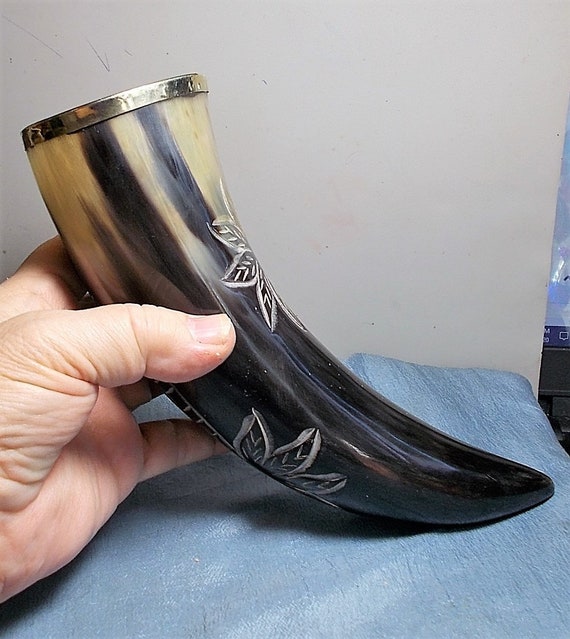In the photograph, a close-up of a Caucasian man's hand is holding a beautifully carved horn, reminiscent of a Viking drinking or blowing horn. The horn, shaped somewhat like a cornucopia, features intricate decorations. Two white flowers with leaves are etched into the horn, enhancing its aesthetic appeal. The horn's color transitions from pale yellow to deep brown as it curves towards the pointed end. A metallic ring, possibly silver or brass, encircles the mouth of the horn, adding a touch of refinement. The artifact rests on a blue cloth, with a creamy white background providing a contrast that highlights the horn’s details.